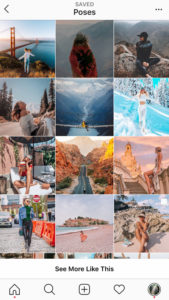This image is a screenshot of someone's "Saved" photos section on Instagram, framed by white borders at the top and bottom. At the top left corner, there's a back arrow, and at the top center, the label "Saved" is prominently displayed. In the bottom section, there is an option to "See More Like This." The central area of the screenshot showcases a grid of twelve saved images, organized in four rows of three pictures each.

- **Top Row:** 
  - The first image features a person posing next to what appears to be the iconic Golden Gate Bridge.
  - The second image captures a person standing amidst a mountainous landscape.
  - The third photo depicts a person sitting in what seems to be a serene mountain setting.

- **Second Row:**
  - The first picture shows a woman seated in a lush forest area.
  - The second photo presents another mountainous scene.
  - The third image features a woman standing in the snow.

- **Third Row:**
  - The first image is of a woman lounging on a unique chair.
  - The second photo showcases a picturesque, winding road.
  - The third image depicts a woman sitting on a set of steps.

- **Bottom Row:**
  - The first picture captures a woman walking down a bustling street.
  - The second photo shows someone enjoying a day on the beach.
  - The last image is of a person standing in front of some rocks on a beach-like area.